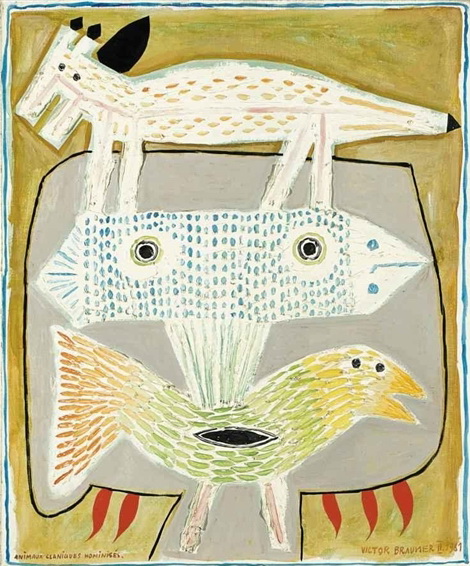This is an intricate and surreal artwork by Victor Brawner, rendered in a hand-drawn, hand-painted watercolor style, featuring an abstract composition with a butterscotch brown, greenish-brown background. Dominating the upper part of the image is a mystical four-legged creature resembling either a dog or a reptile, with white fur or skin accented by small orange scales, black ears, and black eyes. This creature stands atop a hexagon-shaped figure adorned with a white background filled with blue spots and dashes, with central black eyes giving it a peculiar semblance to a fish.

Below this hexagonal figure, there is a striking yellow, green, and brown bird, impaled from the back by a rectangular beak, which appears to stem from the hexagonal form above. The bird features multiple eyes, one on the right side and another embodied in its black wing, resembling an eyeball shape. Around the bird is a subtle gray outline, and red flame-like designs descend on the sides of the hexagon.

In the bottom right corner of the painting, the artist's name, Victor Brawner, is inscribed, indicating the creator of this bizarre and captivating work. The artwork is rich in abstract detail and an Egyptian-like aesthetic, merging various animal forms into a single, cohesive, yet surreal scene.